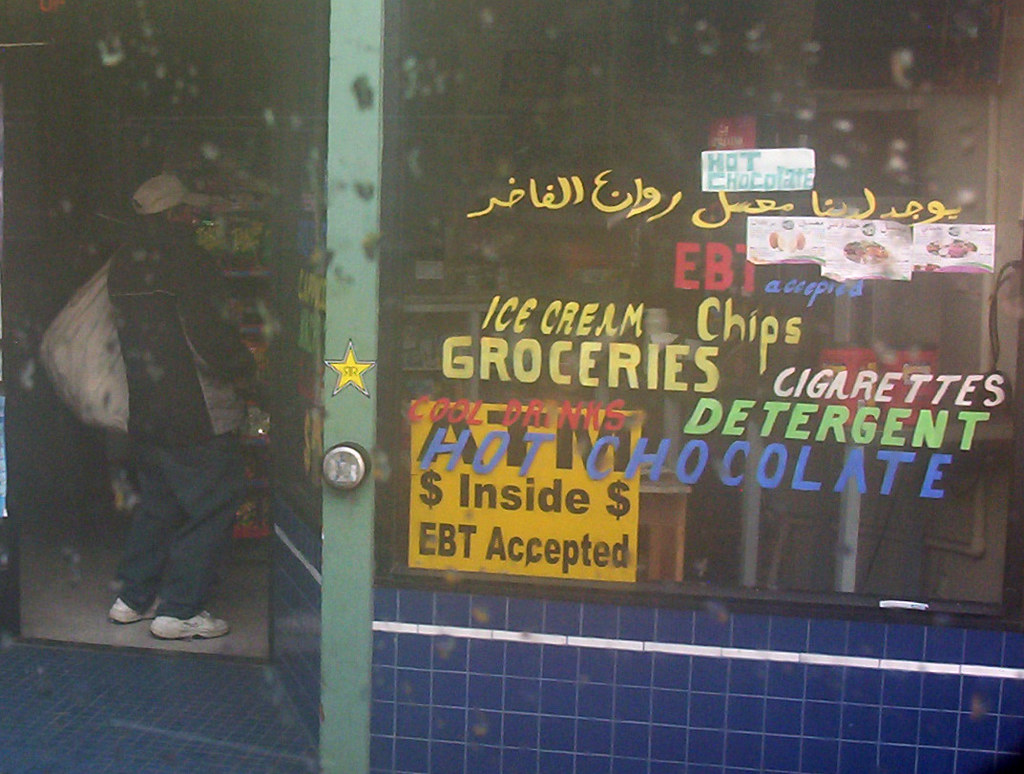The photograph depicts the front entrance of a small, unassuming convenience store. On the left side, the open door reveals a man standing in the doorway. He is dressed in a winter coat, blue jeans, and a white baseball cap, carrying a large white sack slung over one shoulder. To the right of the door, the shop window is adorned with a vibrant array of painted text in various colors, displaying products and services available inside. The text includes both Arabic characters and English phrases such as "EBT accepted," "ice cream," "chips," "groceries," "cigarettes," "detergent," "hot chocolate," and "cool drinks." Among these, a distinct yellow sign with black text stating "ATM inside, EBT accepted" hangs prominently. Below the window, the bottom portion of the shop's exterior is lined with blue tiles. A green pillar is also visible, contributing to the eclectic color scheme of the storefront.